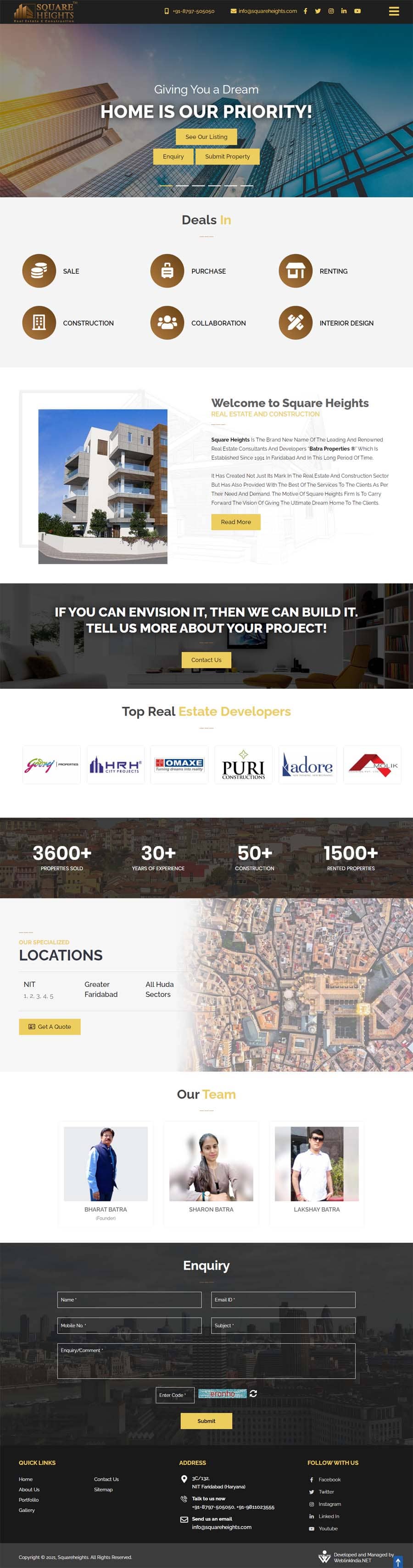The image depicts the homepage of a real estate or construction company's website. At the top of the page, there is a photograph taken from street level, looking up at three towering skyscrapers against the sky. Superimposed on the image is a motivational slogan in bold white font stating, "Giving you a dream home is our priority." Below this image, the design features three yellow rectangles arranged in a triangular formation with one at the top and two at the bottom. 

Further down the page, there is a section labeled "Deals," featuring six brown solid squares arranged in two rows of three. Each square contains a distinct icon: the top left icon depicts coins, the top middle icon shows a shopping bag, the top right icon features a house, the bottom left icon resembles a piece of paper, and the others are indiscernible from the image. 

A header titled "Collaboration" is also visible but accompanied by text that is too small to read clearly. The page welcomes visitors with "Welcome to Square Heights," suggesting that the company specializes in constructing high-rise apartments or industrial-style residences. The page also includes a black triangle with an inspirational tagline: "If you can envision it, then we can build it." The webpage invites users to share their project ideas, positioning itself as a platform for a home builder or general building services.